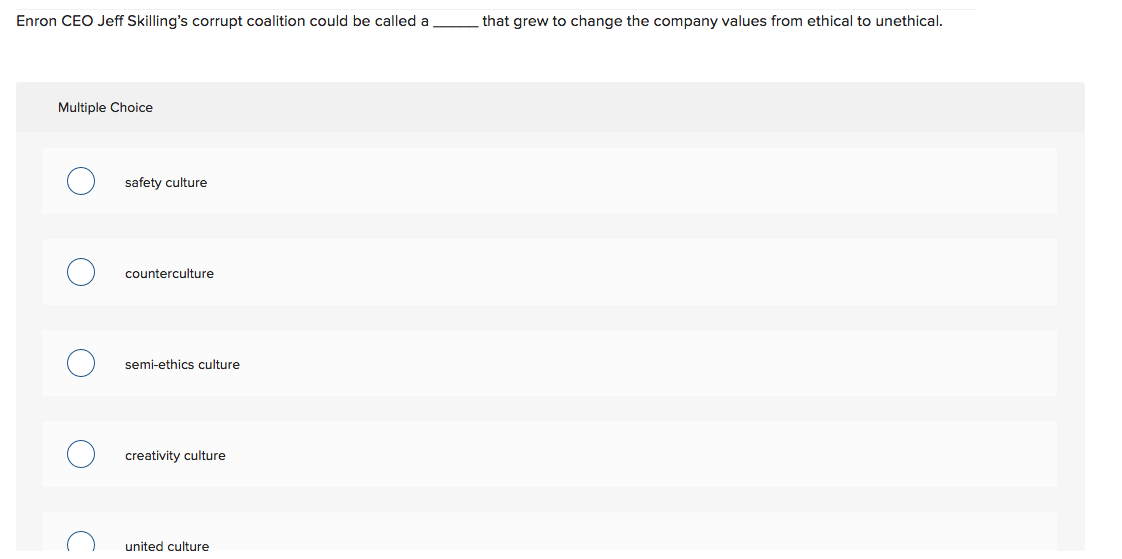The screenshot depicts a minimalist interface, possibly from a laptop or desktop computer, featuring a multiple-choice question. The question, displayed in small black text at the top, reads: "Enron CEO Jeff Skilling's corrupt coalition could be called a ________ that grew to change the company values from ethical to unethical." Below this, the multiple-choice options are presented in a vertical list. Each option—'safety culture,' 'counterculture,' 'semi ethics culture,' 'creativity culture,' and 'united culture'—is encased in a light gray box, with unselected bullet points to the left of each entry. These boxes are set against a slightly darker gray background. Above the options, a label reads "Multiple Choice." The overall layout is simple and uncluttered, characterized by a plain white background and small text that may be challenging for some to read. No photos or illustrations are present. The image captures a straightforward and functional design, consistent with educational or testing software.